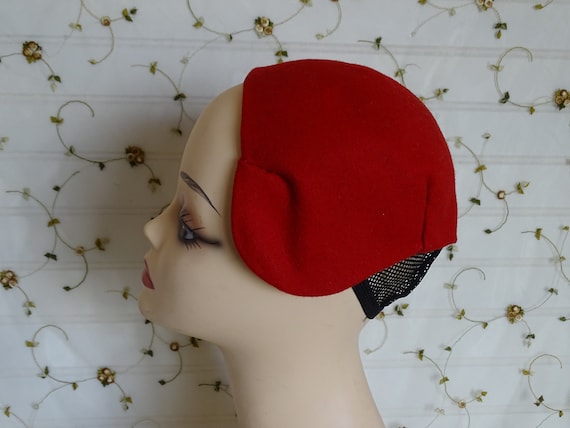This photograph features a detailed side view of a female Caucasian mannequin head set against a backdrop of white with horizontal gray stripes. The backdrop is adorned with a delicate dark green vine design featuring tiny leaves and clusters of white and pink flowers. The mannequin has a smooth, light flesh-colored complexion with exaggerated makeup, including dark black eyeliner, brown eyeshadow, red lips, brown arched eyebrows, and painted long black lashes. The head is turned to the left, showcasing its sharply painted features and small nose.

The mannequin is adorned with a unique red fabric cap that drapes softly over the head, covering the ear area and forming gentle creases. This cap may be made of a felt-like or suede material, adding to its vintage charm. Peeking out from underneath the cap at the back is a black fishnet wig cap, which secures the red fabric cap snugly to the head. The combination of the vibrant red cap and the subtle black mesh adds a touch of texture and contrast to the mannequin's appearance.